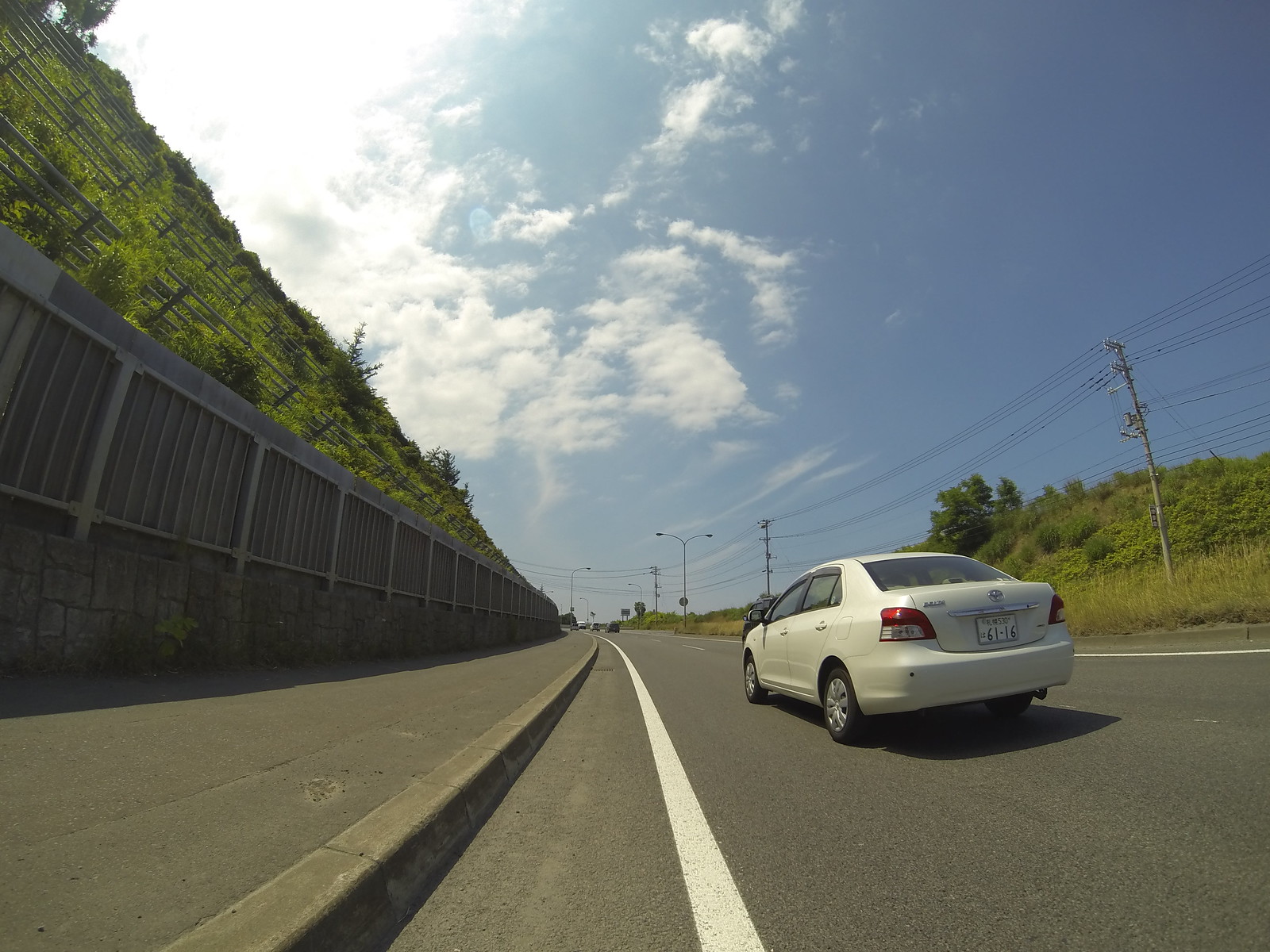A white, four-door Toyota, likely a model from around 2010 or 2011, is captured driving on the left side of a road, indicating a non-American setting. The vehicle is shown from an angle that reveals both its back and side as it moves in a single direction. The scene is set during the daytime, under a sky filled with clouds through which sunlight faintly filters. The surrounding landscape features sparse vegetation, with numerous bushes and a notable absence of trees.